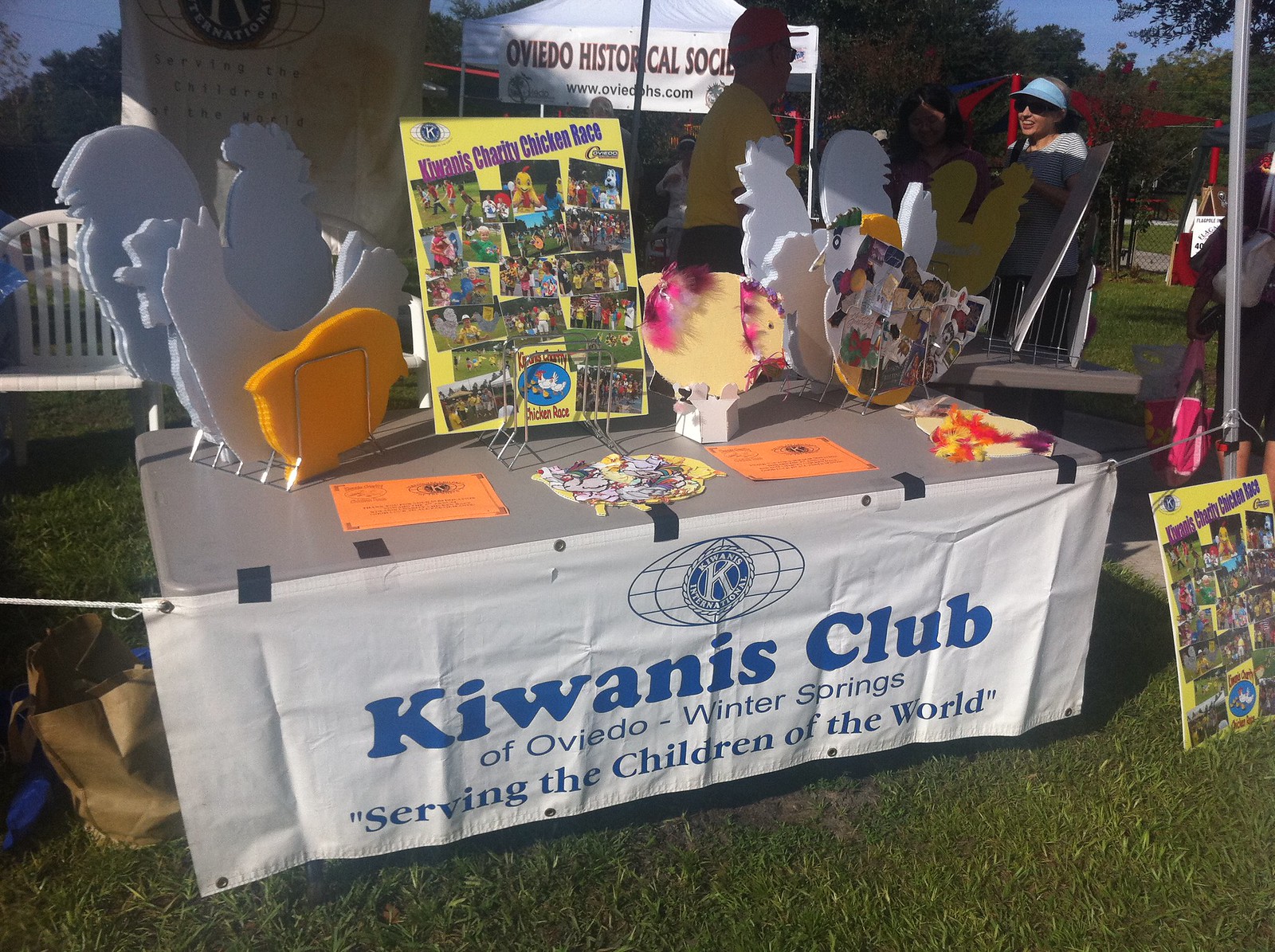The photo captures an outdoor job fair booth for the Kiwanis Club of Oviedo-Winter Springs. The setup is on a grassy lawn, with trees visible in the distant background. The booth features a gray-topped table with a white apron displaying blue text that reads "Kiwanis Club" in large font, followed by "Oviedo-Winter Springs" in smaller font, and a motto: "Serving the Children of the World." A prominent global logo with a 'K' is also visible.

On top of the table, there is a notable poster on an easel advertising the "Kiwanis Charity Chicken Race." This poster includes an array of photos, some featuring chickens. Also on the table are large cutouts of chickens, roosters, and chicks, approximately ten times their real-life size. Various paperwork is scattered across the table's surface.

In the background, another nearby tent is labeled "Oviedo Historical," with people standing around and chatting, adding to the community atmosphere of the event.